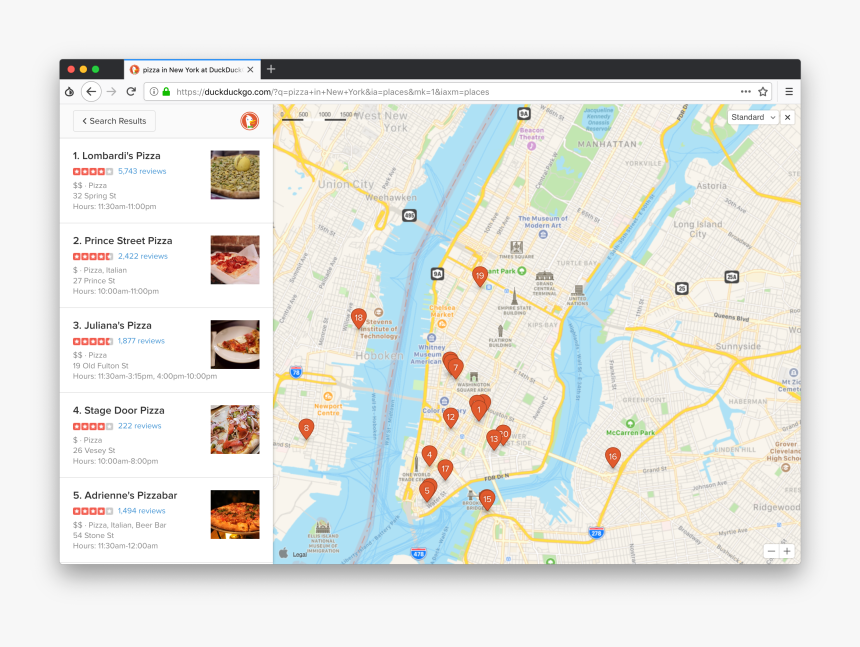The image depicts a search result page on DuckDuckGo.com, where someone has looked up "pizza in New York." The interface resembles that of Yelp, and the page showcases top pizza places in New York with their respective ratings. The first result is Lombardi's Pizza, boasting a 4-star review. Following that, Prince Street Pizza and Juliana's Pizza each have impressive 4.5-star reviews. Stage Door Pizza and Adrienne's Pizza Bar both hold 4-star reviews. On the right side of the page, there is a map displaying orange markers, each shaped like an upside-down teardrop and labeled with numbers. These markers correspond to the numbered list of pizza places, providing a visual representation of their locations within New York City.